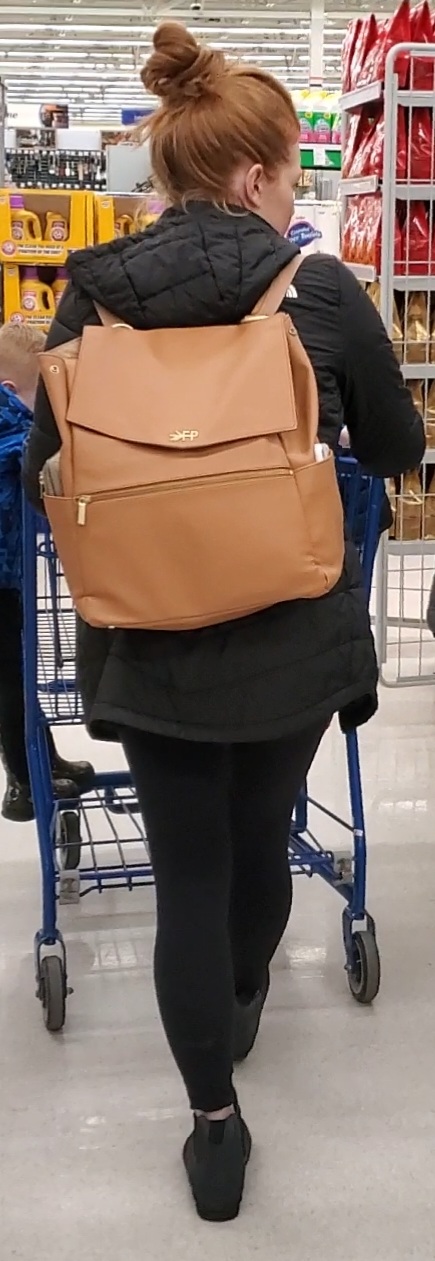In the image, there is a woman and a small child shopping in a store, likely Walmart. The image, taken from the back, showcases the woman, who has auburn red hair tied up in a bun. She is dressed in a black quilted winter jacket with a hood, black yoga pants, and black shoes. The woman carries an elegant brown leather-like backpack with the initials "FP" on it. Pushing a blue shopping cart filled with various products, she navigates through an aisle lined with yellow boxes of laundry detergent. The child, approximately five years old, is standing in the shopping cart, indicating they are likely the woman's. The store floor is a marble white, and racks with red bags of chips and other items are visible in the background, under a striped ceiling. Only a small portion of the child's profile is visible from the side of the cart.